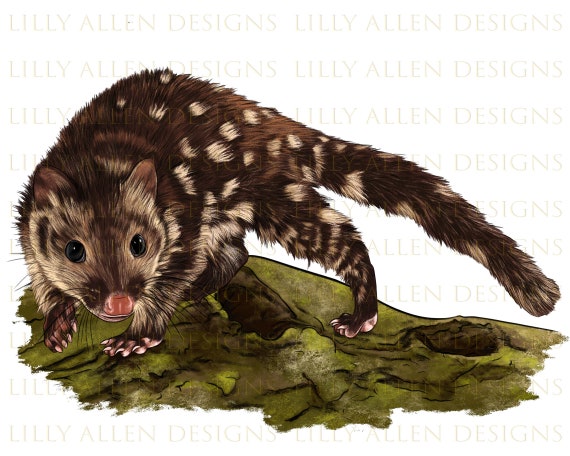The image is a color-illustrated landscape orientation featuring a quoll-like or possum-like creature. The animal, characterized by its elongated, slightly arched body and long tail, is predominantly dark brown with distinguished cream-colored spots. Its face, pointed at the snout, displays a beige and brown color pattern with small, rounded ears. The creature’s posture, facing the viewer, highlights its heavier claws with notably short front paws and longer back paws, positioned low to the ground. The background displays a dark green field dotted with moss-covered rocks, with the watermark "Lily Allen Designs" subtly incorporated in a light yellow hue across the backdrop. Despite the white overall background, the detailed illustration brings the focal rodent-like animal to life, making it appear agile and possibly part of a hypothetical game or narrative setting.